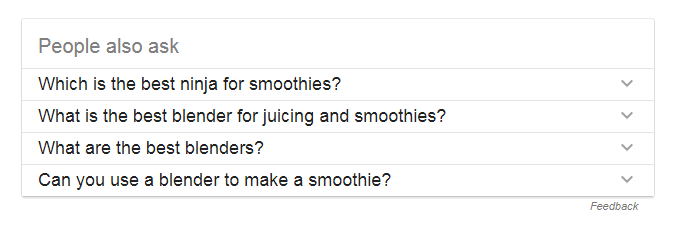The image is a screenshot from a search engine results page, featuring a "People Also Ask" section. The background is completely white, with a central, smaller rectangular white box outlined in light gray. Within this box, there are horizontal lines separating sentences, all in the same light gray. 

At the top of the box, slightly wider than the rest, is the heading "People Also Ask" in a larger, lighter gray font. Below this heading are four individual question boxes, each with its own separate line and distinct gray border. The questions listed are:
1. "Which is the best ninja for smoothies?"
2. "What is the best blender for juicing and smoothies?"
3. "What are the best blenders?"
4. "Can you use a blender to make a smoothie?"

To the right of each question is a clickable arrow icon resembling a 'V'. At the very bottom of the rectangular box, in smaller gray italic font, the word "Feedback" is displayed.